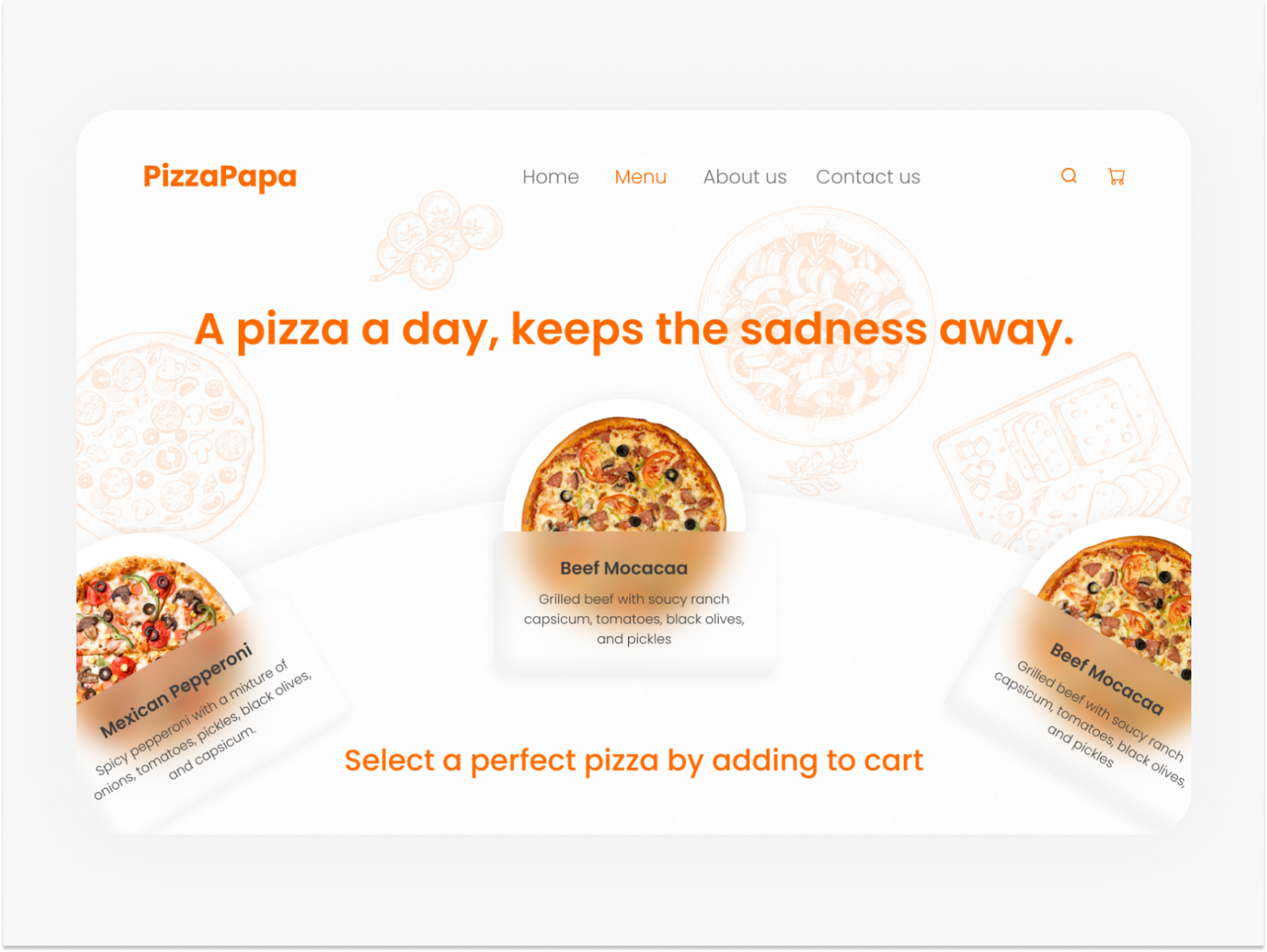This is an image showcasing the website for Pizza Papa. The layout features four primary tabs: Home, Menu, About Us, and Contact Us, with the Menu tab highlighted in orange. Prominently, the site displays the phrase "A pizza a day keeps the sadness away" in the same bright orange. Icons for search and shopping cart functions also share this color theme.

The website's background is predominantly white with simple gray outlines of various pizza types. In the visual, three distinct pizzas are displayed. The first two pizzas, Mexican Pepperoni and Beef Machaca, are presented identically, both topped with their respective ingredients. Descriptions of these pizzas are provided beneath each image. Each pizza is illustrated atop a minimalist tray of cheese with a cluster of tomatoes nearby. Additionally, there is a slightly blurry rectangle overlay on each pizza image, accompanied by an out-of-focus depiction of a woman in the background, suggesting a thematic or narrative element.